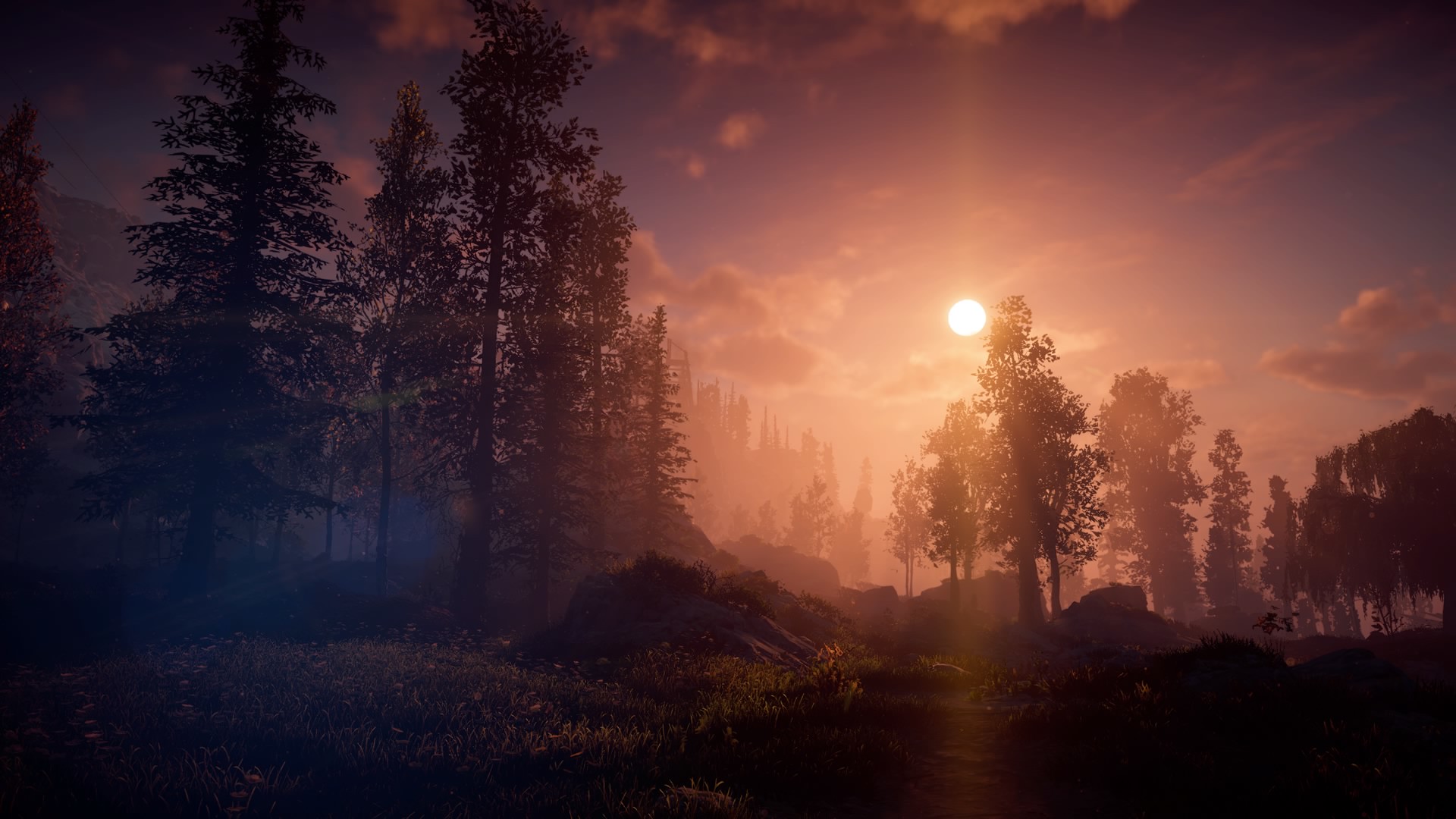A stunning landscape at dusk, showcasing the sun as it prepares to set, casting a warm yet fleeting glow over the scene. The sun hovers just above the treeline, partially obscured but still emitting a soft, golden light. On the left side of the image, an array of tall trees stretches skyward, towering over the shorter trees on the right. The forest appears to nestle in a valley, with varying tree heights creating a textured, layered effect against the twilight sky. The trees in the background seem so tall that they almost touch the scattered clouds above. The overall atmosphere is serene and a bit mysterious, as the encroaching night blends with the remaining daylight in a harmonious balance.